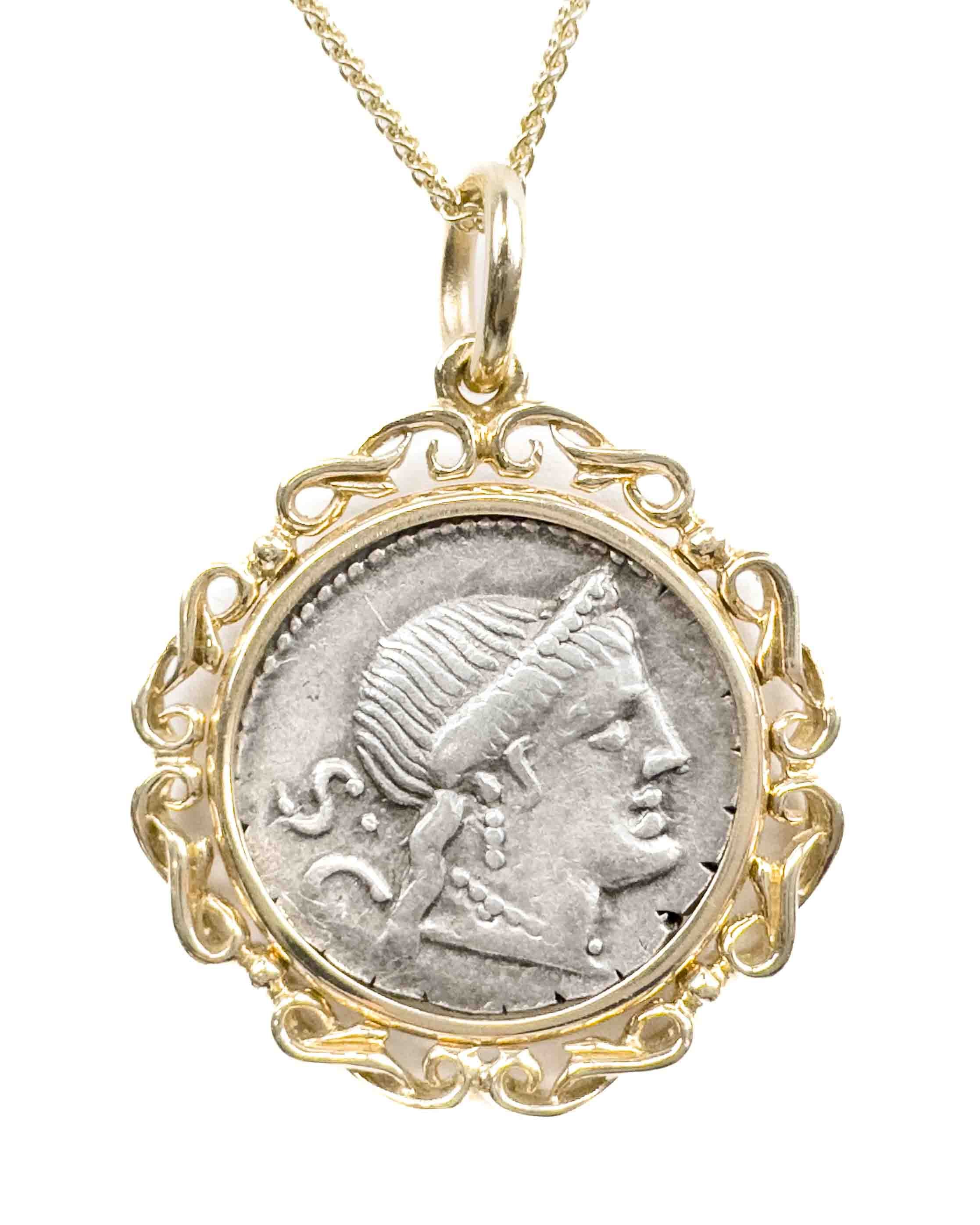This detailed image showcases a gold necklace with a pendant prominently featured against a white background, suggestive of an online marketplace or jewelry website display. Only a portion of the thin, delicate gold chain is visible as it threads through a gold hook that attaches to the pendant. The pendant itself is circular, framed intricately in gold with wavy, ornate carvings. At its center lies an ancient-looking silver coin depicting the profile of a man, possibly an emperor, with distinctive facial features including a pronounced nose and well-defined chin. The man appears to be wearing a cap with hints of hair extending backward. There's an inscription beside the profile, bearing the letters 'S' and 'C'. The pendant's combination of gold and silver, along with its historical design elements, adds to its elegant and timeless appeal.